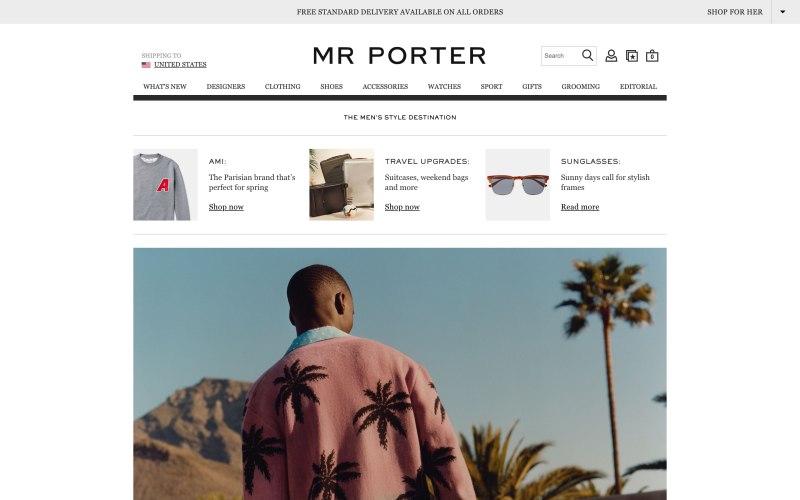**Detailed Description Caption:**

At the very top, in bold and striking text, it reads "Very Great." Below it, there's a banner announcing "Free standard delivery available on all orders. Shop now!" The website prominently highlights shipping availability to the United States, with the iconic logo of Mr. Porter prominently displayed.

The search bar is symbolized by a magnifying glass icon, accompanied by a user account icon resembling a head and shirt. Adjacent to these, there's a shopping bag icon and a favorites icon, depicted as a star within a square overlaying another square.

A navigation menu is laid out, offering categories such as "What's New," "Designers," "Clothing & Shoes," "Accessories," "Watches," "Sport," "Guests," "Grooming," and "Editorial." Beneath this is a black bar with the tagline "The Men's Style Destination."

The centerpiece of the page features a grey long-sleeve shirt with a bold red letter 'A' and 'M', described as "The Parisian brand that's perfect for spring. Shop now," with an underline prompting action.

Further down, there's a travel section showcasing upgrades. It includes images of three suitcases, one of which is toppled over, with a caption "Suitcases, Weekend bags & more. Shop now."

Adjacent to this, sunglasses are highlighted under the tagline "Sunny days call for stylish frames," featuring a pair with brown frames and a "Read more" link.

At the center, a vivid picture features a serene blue sky with a palm tree and green leaves. A mountain looms in the background, and prominently displayed is a purple sweater adorned with designs resembling palm leaves, modeled by an individual with short hair.